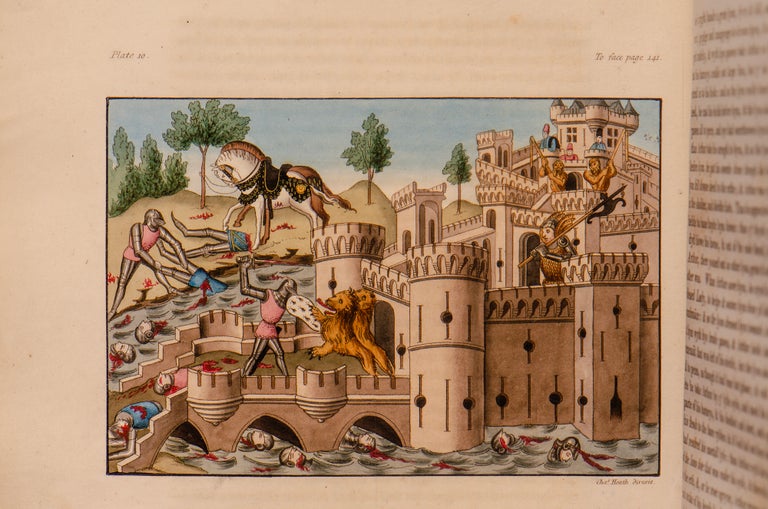This image, taken from a page of an old textbook or picture book, vividly depicts a gruesome medieval battle scene, likely from the Crusades. The annotated page number is uncertain, possibly "Plate 30 or 20" at the top left, while "Too Fair, page 121" is noted at the top right. The detailed painting centers around a large, sandy-colored castle with multiple pillars and walkways, seemingly surrounded by a moat filled with severed, bloodied heads and disembodied limbs.

Inside the castle walls, a chaotic scene unfolds: knights in gold and silver armor stand guard. Outside, knights clad in plate armor with pink cloth coverings clash amid a bloody massacre. Particularly notable is a striking knight in pink armor with a white shield bearing a black pattern, seen battling two lions at the castle gate. The battlefield shows numerous decapitated heads, some still in their helmets, and bloodied soldiers, with blue-shirted knights lying mostly slaughtered.

In the top left, a white horse steps over a disembodied, bloodied man, adjacent to trees on distant hills. Further left, a knight drags a fallen comrade from the water. Amid the melee, one knight is drowning an opponent in the river while another wields a polearm. The right page of the book, out of focus, hints at further context.

This intensely detailed portrayal captures the brutality and chaos of historical warfare, immortalizing a moment of fierce combat and tragedy.